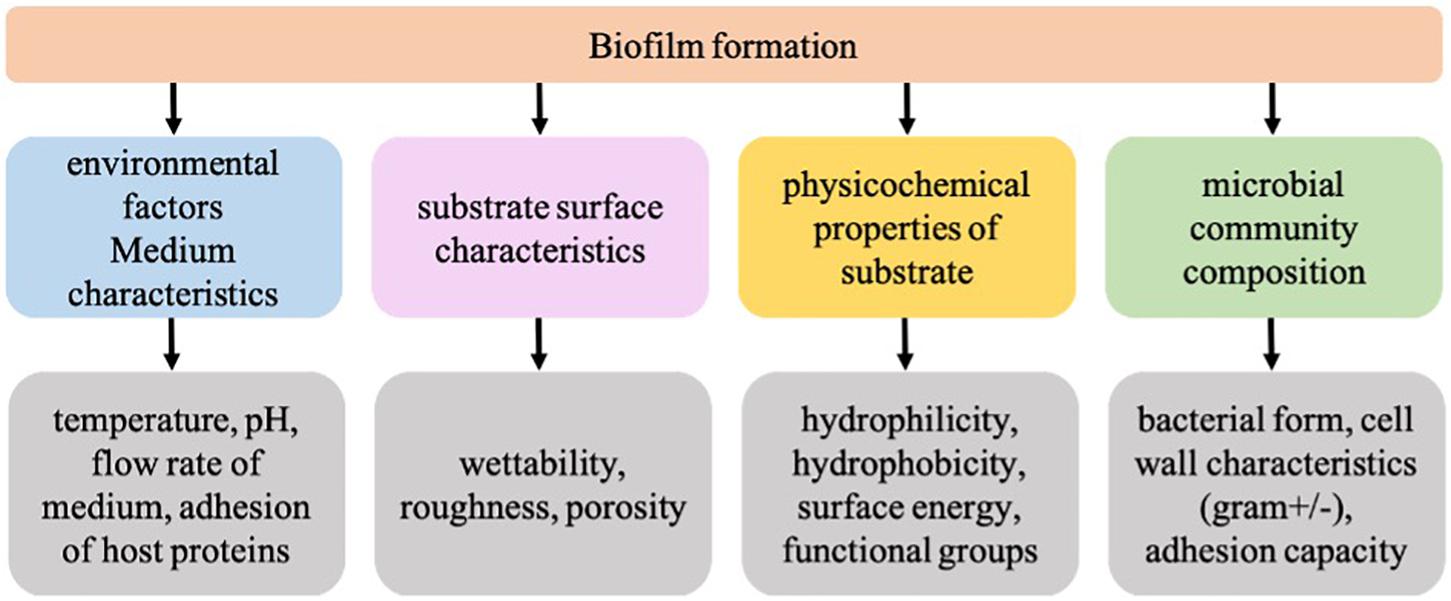The diagram titled "Biofilm Formation" features an organizational chart with a salmon-colored title bar situated at the top of this horizontal image. From this title bar, four black arrows lead downward to four color-coded text boxes: a blue box labeled "Environmental Factors, Medium Characteristics," a lilac box labeled "Substrate Surface Characteristics," a goldenrod yellow box labeled "Physiochemical Properties of Substrate," and a seafoam green box labeled "Microbial Community Composition." Each colored box is further linked by black arrows to a corresponding pale gray text box below. The gray boxes contain detailed elements as follows: the first gray box, connected to the blue box, lists "Temperature, pH, Flow Rate of Medium, Adhesion of Host Proteins"; the second gray box, linked to the lilac box, lists "Wettability, Roughness, Porosity"; the third gray box, paired with the goldenrod yellow box, contains "Hydrophilicity, Hydrophobicity, Surface Energy, Functional Groups"; and the fourth gray box, associated with the seafoam green box, details "Bacterial Form, Cell Wall Characteristics (Gram Positive or Gram Negative), Adhesion Capacity." The overall design utilizes serif black text and pastel colors to create a visually structured flowchart outlining the factors influencing biofilm formation.